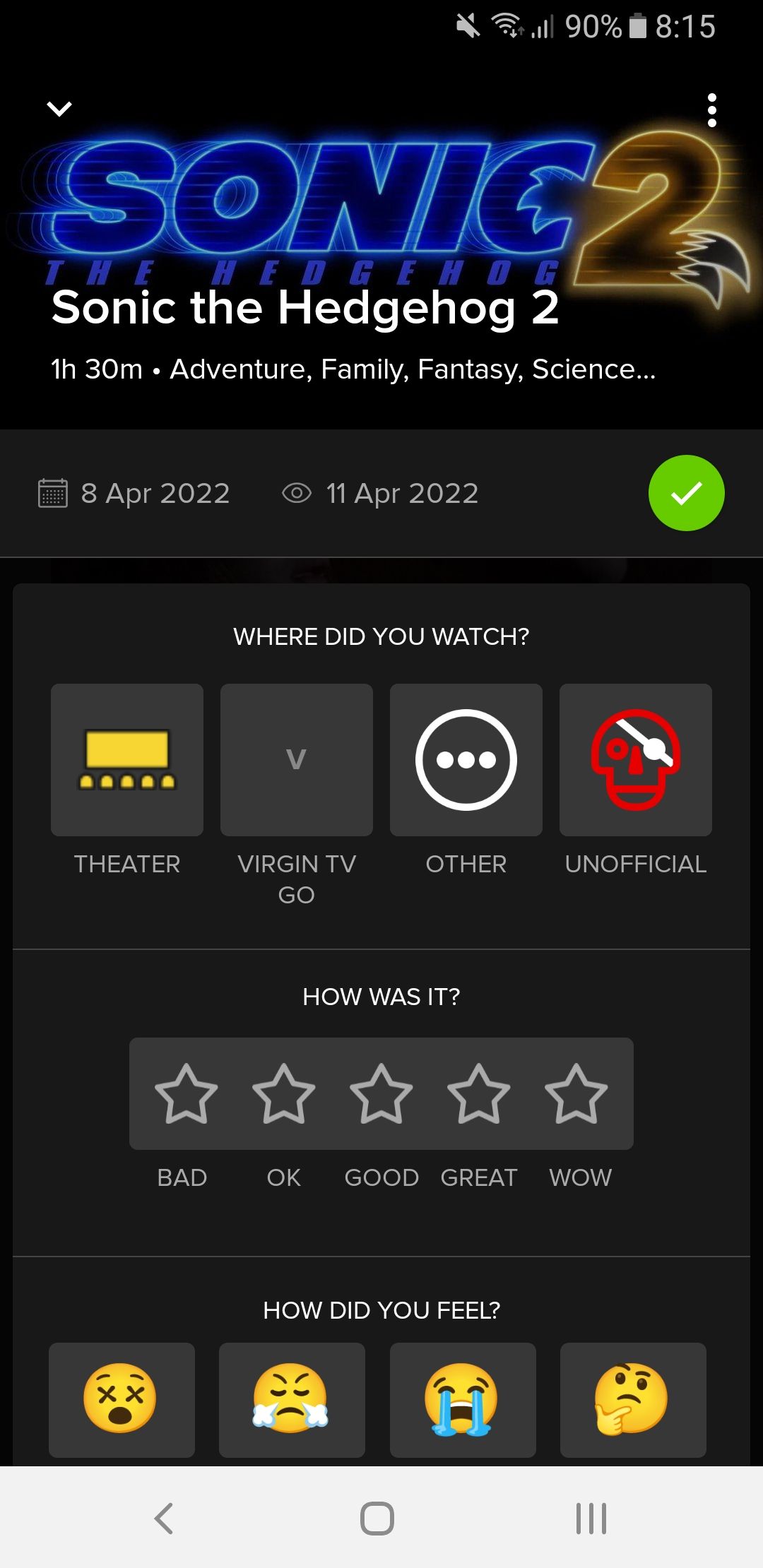A detailed screenshot of an Android cell phone displaying the summary of Sonic the Hedgehog 2 is presented. The screen shows that the movie, listed under adventure, family, fantasy, and science fiction genres, has a runtime of 1 hour and 30 minutes. The movie title, "Sonic the Hedgehog 2," is prominently displayed with "Sonic" in bold blue writing and "2" in white underneath. The movie's release date is noted as April 8th, 2022, and the user watched it on April 11th, 2022. There's a green checkmark indicating the user has completed watching it.

The screen prompts the user with a question, "Where did you watch it?" with selectable options including "Theater," "Virgin Go," "Other," and "Unofficial," illustrated by respective icons. The "Unofficial" option seemingly implies watching a pirated copy. Below this, a 5-star rating system labeled "How was it?" allows the user to rate the movie; the stars represent ratings from "Bad" to "Wow." 

Additionally, there's a "How did you feel?" section featuring emojis to capture the user's feelings about the movie, ranging from a bored or confused face, an angry face, a crying face, to a thoughtful or puzzled face. 

At the bottom of the screenshot, within a gray bar, are the browser navigation controls including "Go back," "Open another tab," and "More options," indicating the image was taken within a web browsing session.